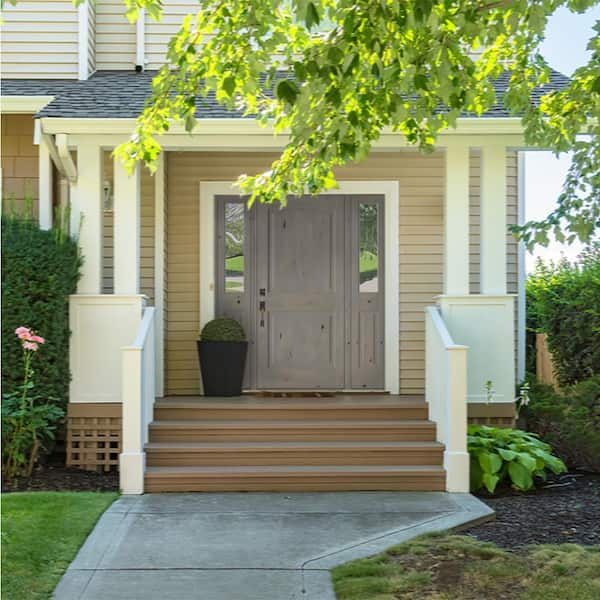This outdoor daytime photograph captures the front facade of a well-kept house. Central to the image is a dark grey front door, flanked by tall, thin windows. The house is constructed of light brown wood paneling, adorned with white trim and decorative elements. Leading up to the door is a short staircase with four light brown steps, complemented by a white banister. These steps ascend to a small porch area, also crafted from light brown wood. A grey walkway extends from the staircase, bordered by patches of green grass and various plants, including a pink flower on the left side. The roof, made of dark grey tiles, slopes down to cover the porch area. The upper portion of the house remains partially hidden by the vibrant green leaves of a tree, visible at the top right of the image, adding to the serene, well-maintained atmosphere of the neighborhood.